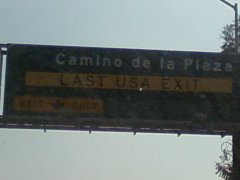This photograph captures what appears to be a highway sign directing drivers to an exit. Due to the small resolution and dim lighting of the image, fine details are difficult to discern. The sign prominently indicates "Camino de la Plaza" at the top. Below this, in a yellow box with all capital letters, it reads "Last USA Exit." Further down on the left side of the sign, another yellow box displays "Exit Only" accompanied by an arrow. The canvas behind the sign is a pale greenish-blue hue, suggesting the sky. Visible on the right side of the image is the support post for the sign, and some tree foliage peeks out from behind it.